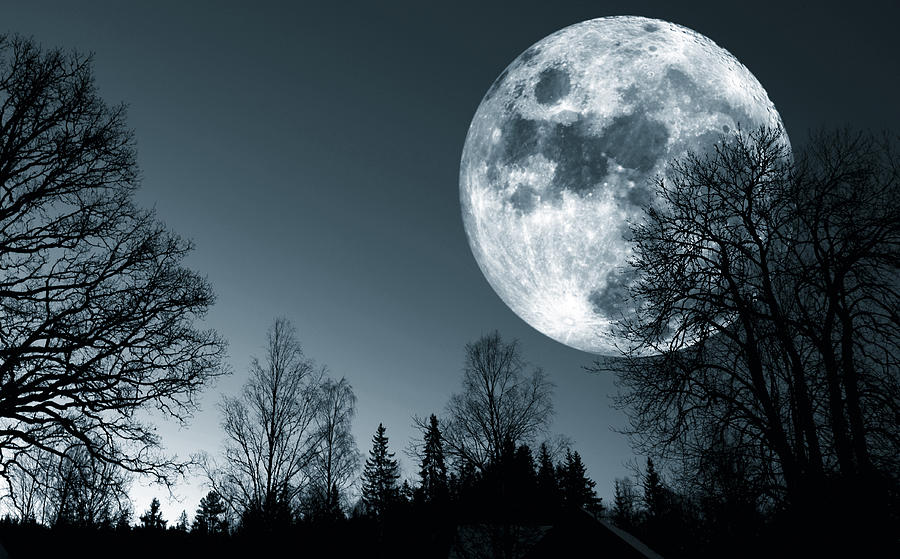In this striking nighttime photograph, the central focus is on an exaggeratedly massive moon that occupies a significant portion of the right side of the image. The moon, rendered in full form, displays intricate shading with stark white areas and contrasting darker patches, giving it a textured appearance. The scene is observed from ground level, where tree branches crisscross the lower quarter of the moon, adding a mystical element to the composition. These branches, likely bare due to the time of year, cast silhouettes against the moon's luminous backdrop. Surrounding the moon, the sky transitions into deep hues of blackish and grayish-blue, enhancing the ethereal atmosphere. In the distance, one can make out the darkened figures of more trees, including evergreens, extending upwards with no signs of human presence or habitation. The overall effect is a mesmerizing, seemingly manipulated vision of nature lit by the oversized celestial body, with just a hint of mysterious illumination rising from the bottom left corner.